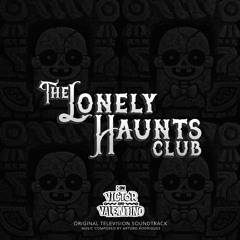The image, likely the cover of an album, is a perfect square with a completely black background. Four barely visible, almost skeletal little girls, shaded in very dark gray, blend seamlessly into this background. In the center, bold white text spans four lines, reading "The Lonely Haunts Club." Toward the bottom, more prominent white text states "Victor Valentino," followed by smaller, lighter gray text that reads "Original Television Soundtrack." Below this subtitle, a barely legible line indicates it was composed by an unnamed individual due to the blurriness. The overall aesthetic is minimalistic yet eerie, fitting a hauntingly mysterious theme.